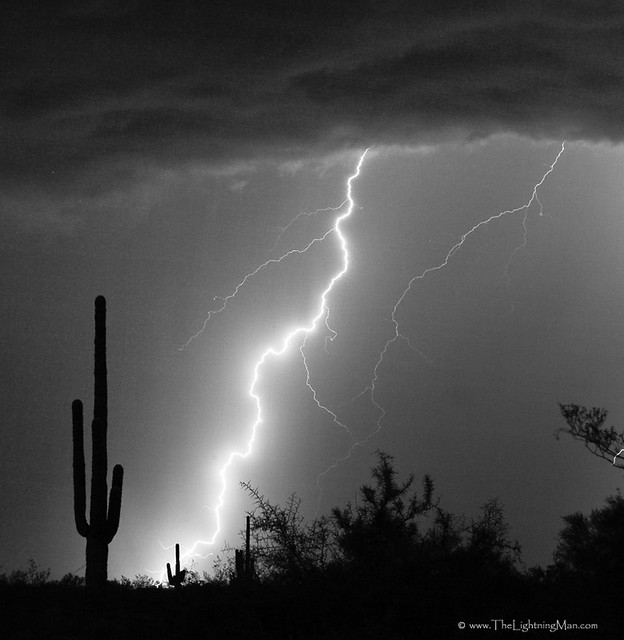This square, black and white photograph captures a dramatic desert thunderstorm at night. Dominating the image is a striking vertical lightning bolt that runs from the top to the bottom of the frame, with smaller branches extending from it. To its right, a thinner, less intense lightning bolt also reaches the ground, creating a dynamic scene. On the ground, we see a series of cacti: a prominent three-pronged cactus stands to the left in the foreground, while two additional cacti of varying sizes and complexity are positioned further into the distance. The scene is set against a dark sky filled with ominous clouds, adding to the overall tension. The image is punctuated by shrubbery and trees at the bottom, offering a rugged, natural contrast to the electrifying sky. The website www.thelightningman.com and a copyright symbol are discreetly printed in the lower right-hand corner.